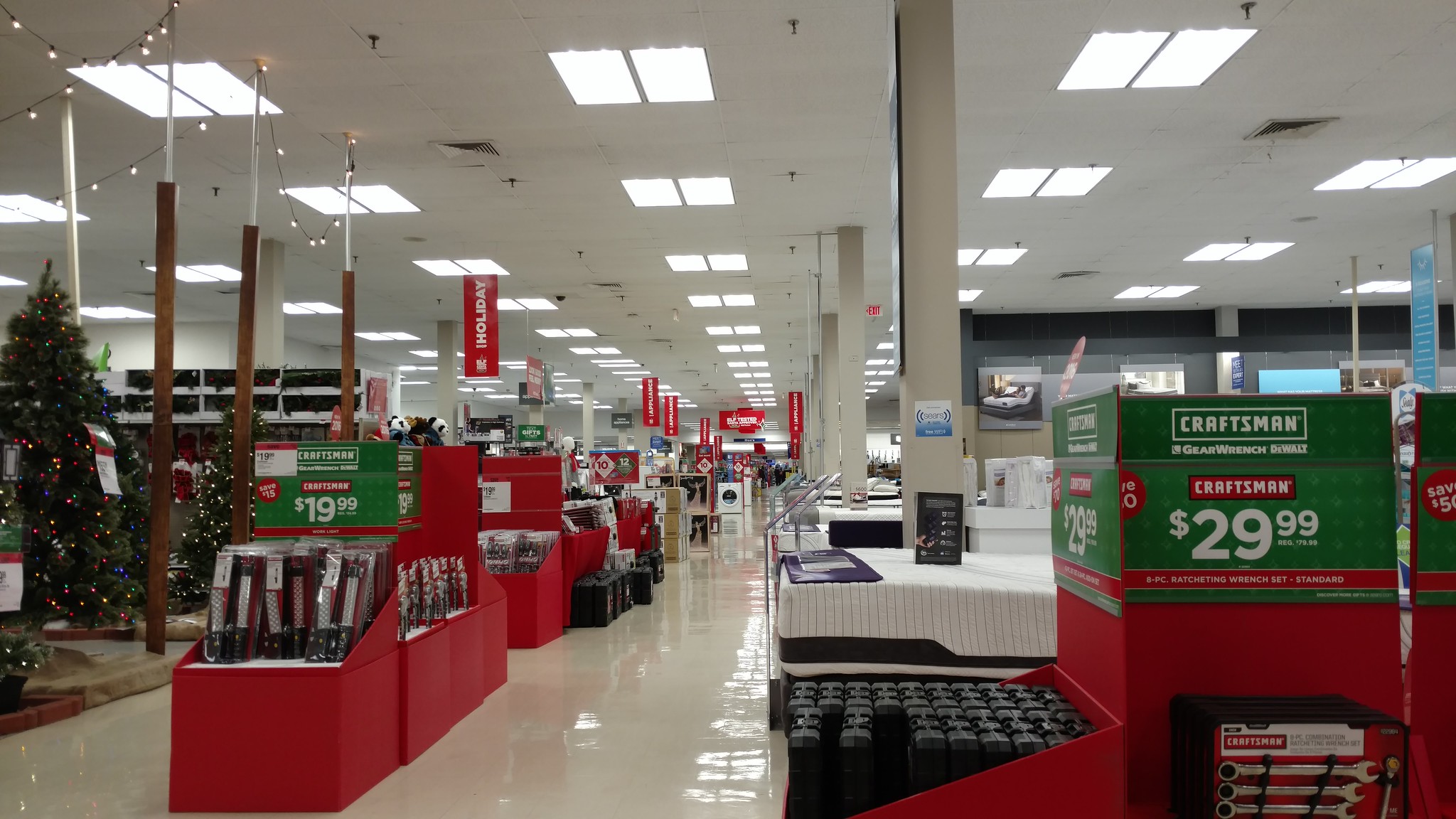This photograph captures the bustling interior of a department store, likely located within a mall. The left side of the image showcases a festive display of decorated Christmas trees available for purchase. Adjacent to this, in the left center of the frame, are several sections featuring tools, with a prominent green sign marking a Craftsman tool set priced at $19.99. These sections of goods continue in a structured manner down the aisle.

To the right of the image, a variety of mattresses and beds are on display, indicating a home goods section. In the bottom right corner, another tool display features an array of toolboxes and wrenches, highlighted by a sign reading $29.99, in Craftsman's signature green, red, and white colors. The white ceilings are lined with numerous rectangular lights, evenly illuminating the entire store layout. This detailed depiction offers a comprehensive view of the diverse range of products and the organized arrangement within the department store.